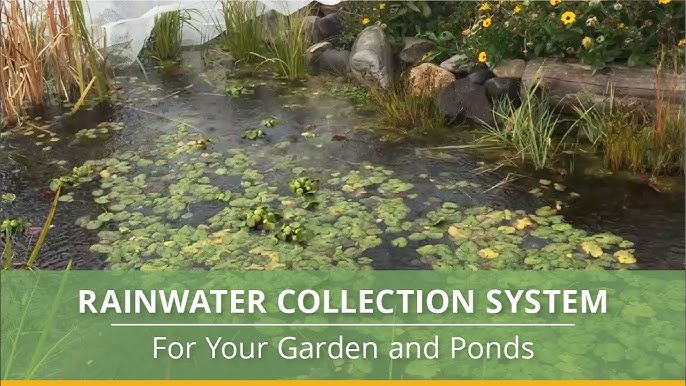The image depicts a tranquil pond with murky water adorned with lily pads. Encircling the pond are tall grasses, interspersed with rocks and a log adding a natural rustic charm. In the top left corner of the image, there is a piece of clear plastic tarp, which seems to be connected to the pond's functionality, possibly as part of a rainwater collection system. The upper right corner showcases a cluster of vibrant yellow flowers amidst a lush bush. A green, semi-transparent banner stretches across the bottom of the image, allowing a view of the pond below. Overlaid on the banner, in white text, is the informative phrase: "Rainwater collection system for your garden and ponds." This suggests that the clear plastic tarp visible in the upper part of the image likely plays a role in this system, although its connection is not immediately clear from the visual provided.